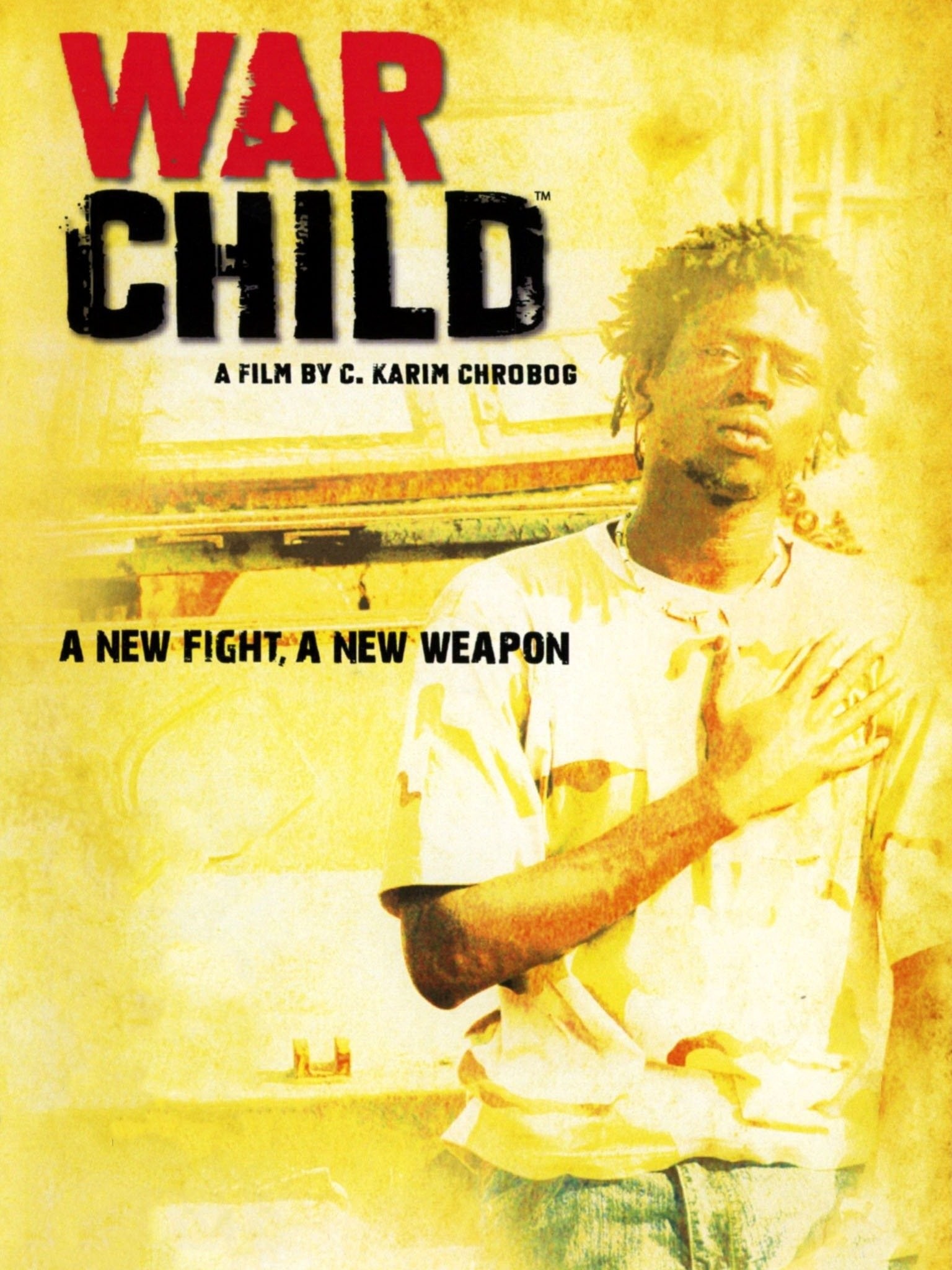This is a detailed caption:

The image depicts a movie poster for a film titled "War Child," prominently displayed in the upper left-hand corner. Directed by C. Connor Karam Charbrooke, the tagline "A New Fight, A New Weapon" hints at the film's intense and possibly action-oriented theme. The poster is predominantly dominated by a striking, vibrant yellow hue that draws immediate attention and largely obscures other elements in the background. In the foreground stands a young Black man, central to the composition, who appears to be the lead character. He is dressed in a white shirt and blue jeans, with his right hand crossed over his chest, resting on his left pectoral, symbolically placed over his heart. The intense color and the character's serious pose suggest emotional depth and a powerful narrative.